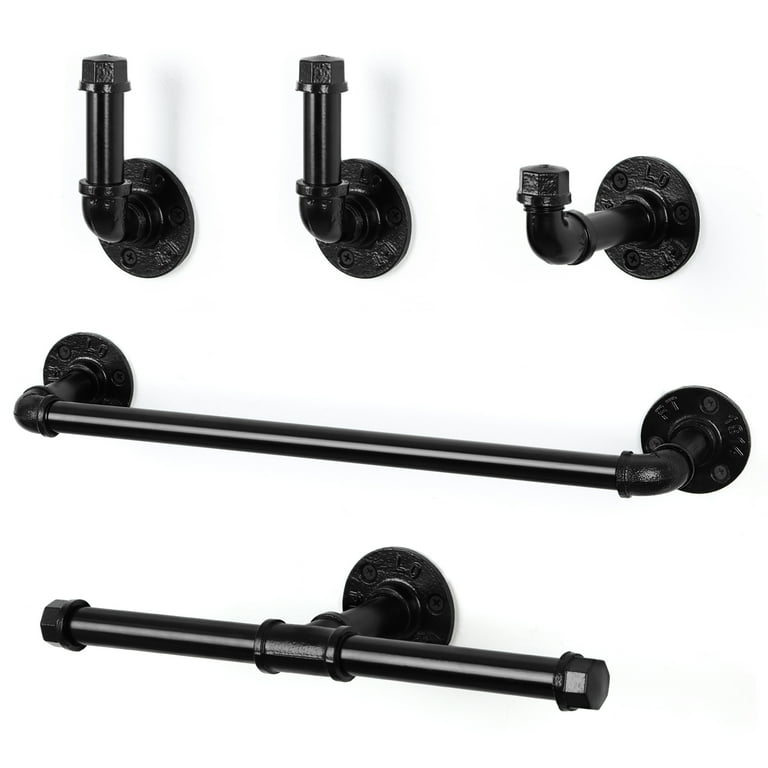The image showcases a display likely intended for a website to feature bathroom hardware products against a white background. The display consists of five black metal fixtures, designed in an industrial style resembling plumbing pipes, flanges, and fittings, all painted and polished in black. At the top of the image, three black pipes extend out from the background and curve upwards, resembling hooks or possibly robe hangers. Below these, a black pipe runs horizontally across the middle, functioning as a towel rack. Underneath this, another black pipe extends horizontally with ends that suggest it could be a toilet paper holder. The overall design incorporates a rustic, repurposed aesthetic with the use of cast metal plumbing elements, adding a unique touch to typical bathroom accessories.